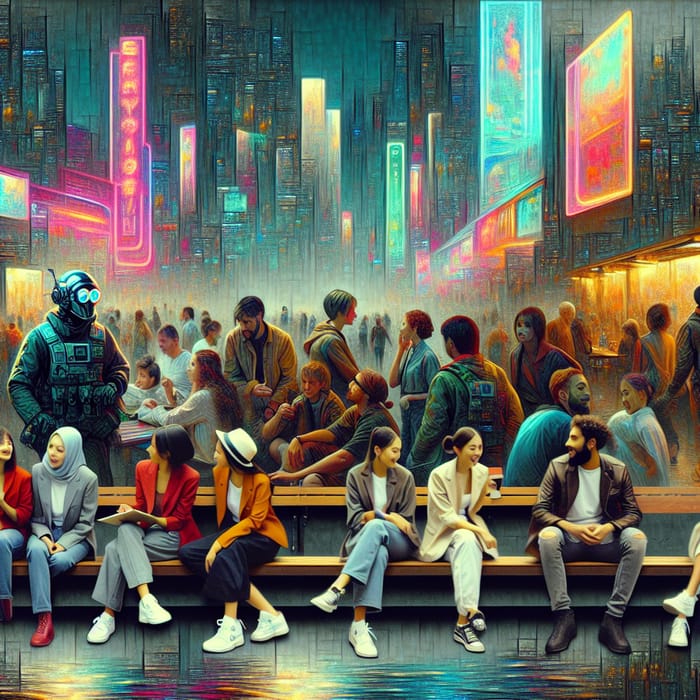The painting depicts a bustling nocturnal scene in Times Square, with a vibrant cityscape drenched in hues of green and yellow, punctuated by neon signs and billboards. Dominating the left side of the composition is a building adorned with various video monitors emitting blues and oranges, all set against the greenish façade. A pink neon sign with yellow letters illuminates the right side, although its text remains indecipherable.

In the foreground, a wooden bench serves as a gathering point for approximately 20 individuals, mostly young people engaged in conversations. Their diverse attire includes colorful jackets, hats, and even a hijab. Among them, a striking figure dressed in a space-cop-like outfit catches the eye; his ensemble features a gas mask with glowing blue eyes, a metallic chest guard, and a substantial headset, evoking a futuristic or military aesthetic.

Adjacent to this bench, two women in red and orange jackets look skyward, seemingly captivated by something above, with only dangling feet of unknown individuals visible, hinting they might be hovering or on a higher level. The street behind them is teeming with more people, creating a bustling, almost chaotic atmosphere. The crowd extends into the misty distance, where high-rise buildings and neon billboards in teal, purple, pink, and orange fade into a pastel-colored haze, underscoring the depth and dynamism of the city at night.